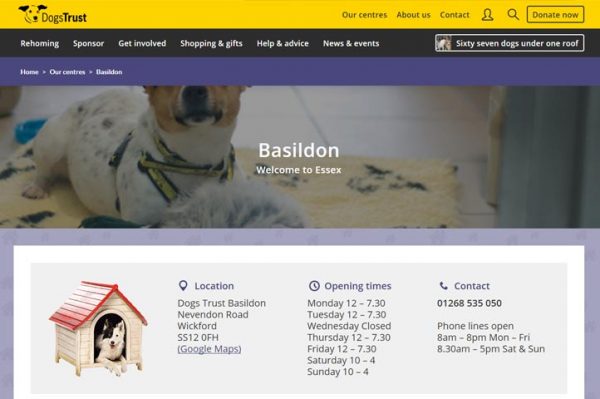This image showcases the Dogs Trust Basildon website's homepage. The navigation menu features categories including "About Us," "Contact Us," "Donate Now," "Links," "Rehoming," "Sponsor," "Get Involved," "Shopping and Gifts," "Help and Advice," and "News and Events." The website prominently mentions that they have 67 dogs currently under their care. The shelter is located under one roof at Nevendon Road, Wakeford, Basildon, Essex, SS12 0FH. The location can be viewed on Google Maps for convenience. Additionally, the shelter's opening hours are listed, specifying they are open on Mondays from 12:00 PM to 7:30 PM.